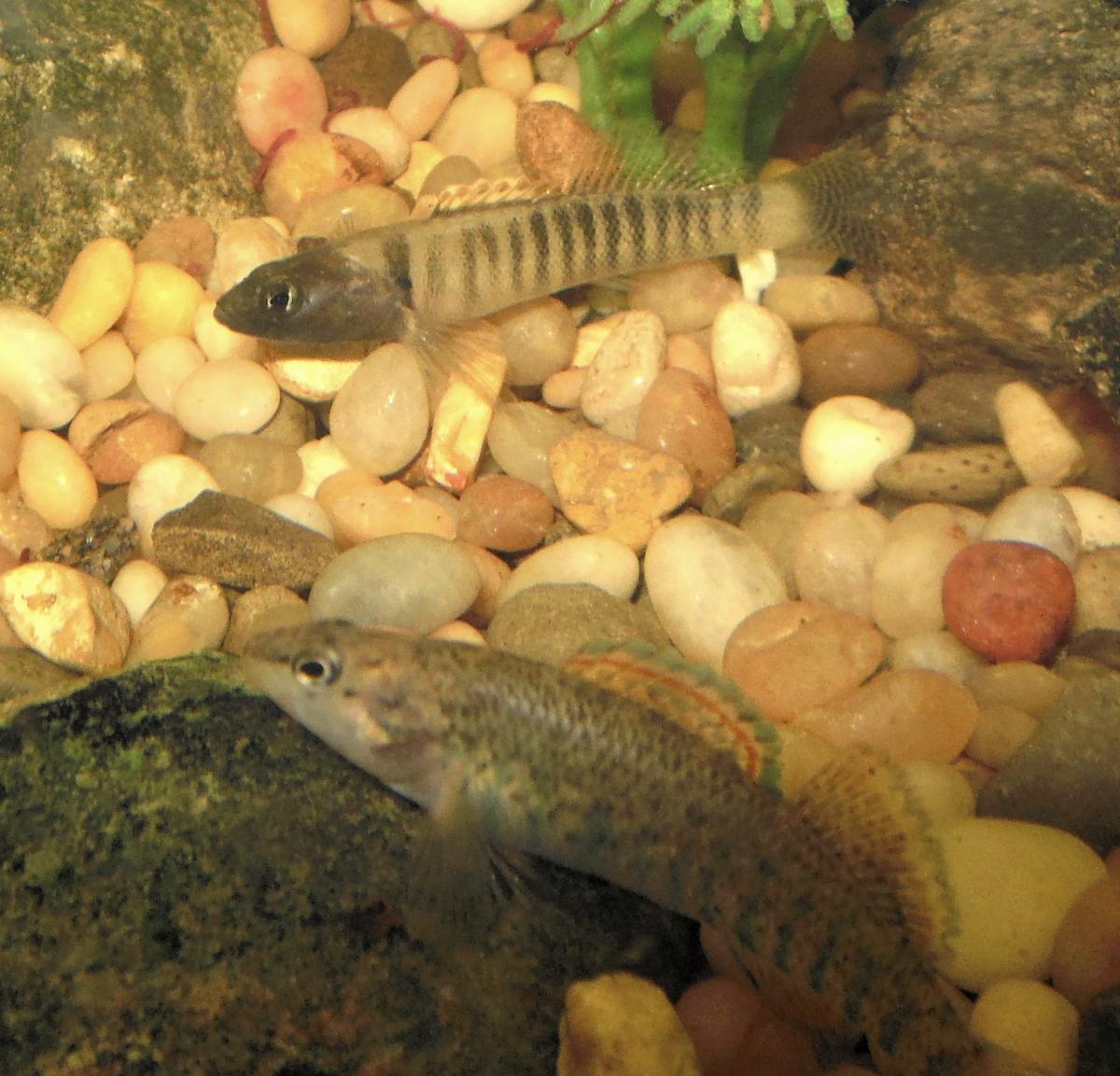This detailed photograph captures two fish swimming underwater against a vibrant, pebble-strewn floor. The water is so crystal clear that it appears almost invisible, making the stones and pebbles on the bottom prominently visible. These pebbles vary in color, ranging from light pink, light orange, green, white, grey, to brown, and are mostly round in shape. Larger, dark green stones are also scattered throughout the scene. 

The two fish, each about four inches long, exhibit distinctive features. The first fish has a dark grey head, transparent fins positioned right behind its gills, and a tan body adorned with vertical black stripes extending to its speckled tail. The other fish showcases a body speckled in green and brown, a pinkish head with a white underside, and a striking blue dorsal fin accentuated by a red stripe.

Both fish appear alert, with open eyes, engaged with their surroundings, and are captured swimming towards the left side of the image. This underwater scene, potentially set in an aquarium, offers a rich display of colors and textures, harmonizing the natural allure of aquatic life.